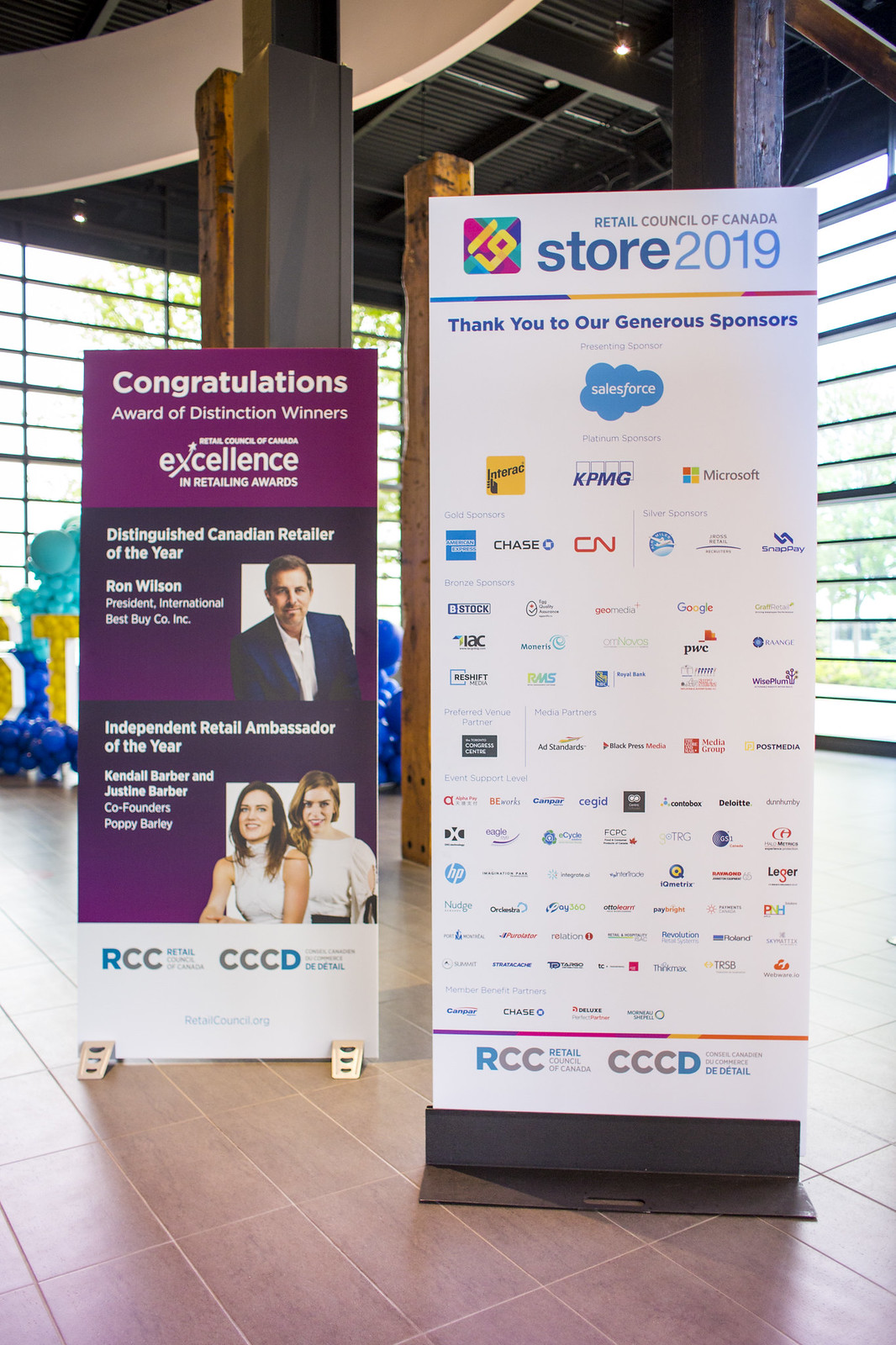The image depicts a corner inside a contemporary display room, characterized by its high-quality tiles, absolutely enormous windows, and a very well-lit ambiance filled with natural light filtering through the windows that form the walls. The space is modern, incorporating large reclaimed wood beams that merge seamlessly with its sophisticated architecture. In this elegantly illuminated room, where the light casts subtle shadows towards the camera’s point of view, stand two tall placards positioned against large columns that stretch up to the high ceiling.

The placard in the foreground on the right has a white background and carries the title "Retail Council of Canada Store 2019." It showcases a plethora of sponsor logos under the heading "Thank you to our generous sponsors," highlighting various tiers of sponsors: Salesforce as the presenting sponsor, with Platinum sponsors including Interac, KPMG, and Microsoft, and Gold sponsors like American Express, Chase, and CN, among others in Silver, Bronze, and event support levels.

The placard on the left acknowledges achievers with the title "Congratulations, Award of Distinction winners, Retail Council of Canada Excellence in Retailing Awards." It features profiles such as the Distinguished Canadian Retailer of the Year, Ron Wilson, President of International Best Buy Company, Incorporated, and the Independent Retail Ambassadors of the Year, Kendall Barber and Justine Barber, co-founders of Poppy Barley. This sophisticated setting clearly serves as a special venue for such distinguished presentations and acknowledgments.